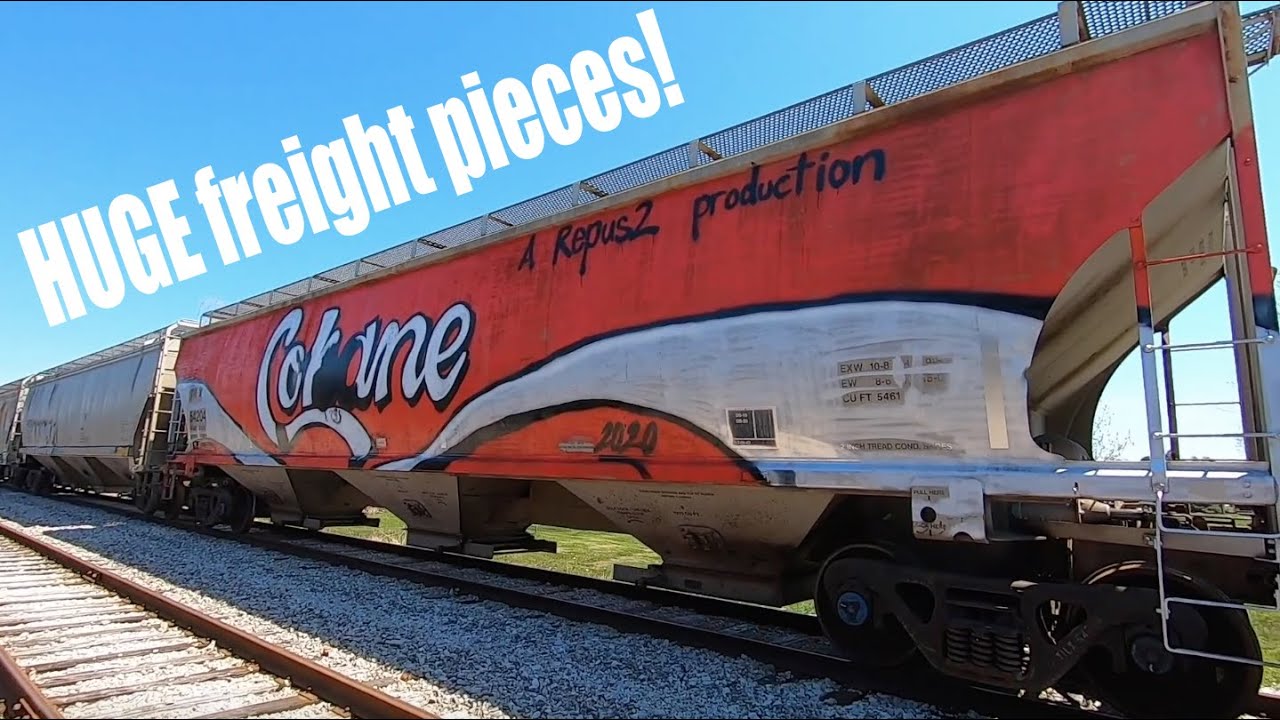The photograph captures a scene at a train yard featuring a three-car train on the further of two railroad tracks, surrounded by white gravel. The focal point of the image is a train with two beige-colored cars at the front, followed by a red and white car designed to mimic the Coca-Cola logo, though it reads "C-O-K-A-N-E." Graffiti or artwork in cursive font, possibly as a statement on production, adorns this car. Above the train, the phrase "Huge Freight Pieces!" is digitally superimposed against a clear blue sky. Black text stating "A Repus 2 Production, 2020" adds a final touch to the image.